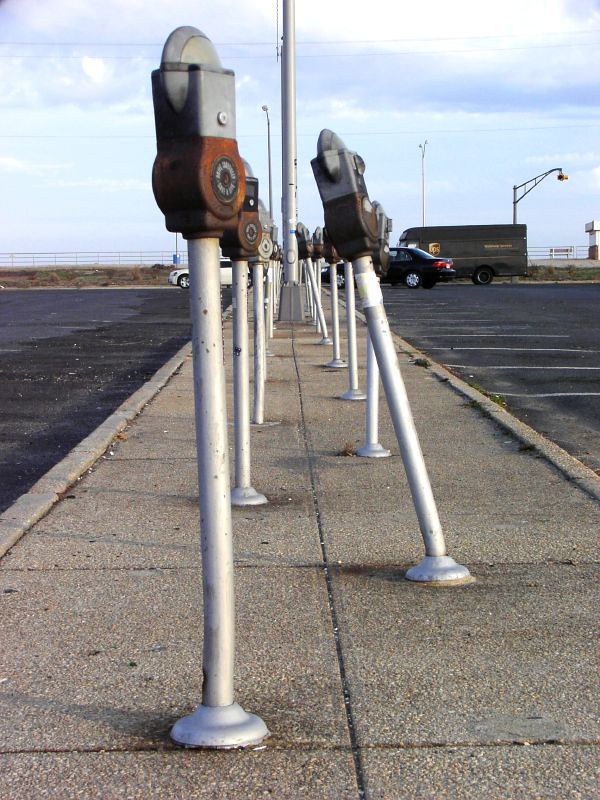The image depicts a black asphalt parking lot with a white-lined parking grid. Down the center of this parking lot runs a whitish-colored sidewalk flanked on both sides by old, rusty, gray parking meters with faded, dirty red bodies mounted on slim silver bases. The meters, arranged in two rows, extend down the length of the sidewalk, although many are leaning forwards or backwards, suggesting disrepair. In the background, a black sedan, a brown UPS truck, and a white car are parked on the right and left sides of the lot respectively. The sky is visible towards the back of the picture, providing a sense of depth to the scene.